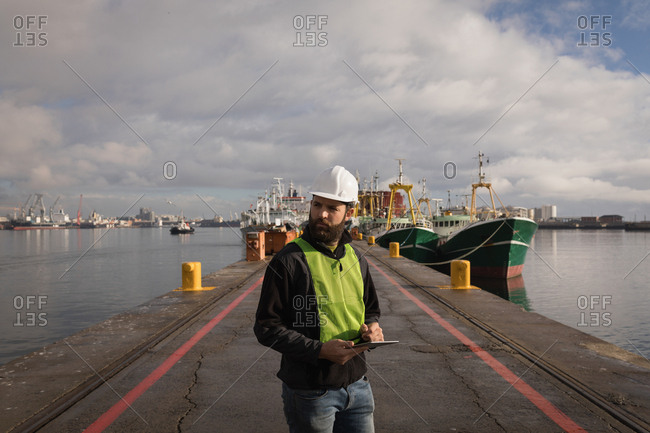A bearded dock worker wearing blue jeans, a black long sleeve shirt, and a yellow reflective safety vest stands on a long pier, which extends into calm waters surrounded by various boats. The man, positioned centrally in the lower half of the image, also wears a white construction hard hat and holds a tablet or clipboard, seemingly taking inventory or overseeing operations with a serious demeanor. To his right, two blue-green ships with white stripes are docked, while smaller, indistinct boats are visible in the distance to his left. Multiple yellow pylons line the pier, serving as mooring points for the vessels. The scene takes place under a daytime sky filled with white, puffy clouds, and a distant city skyline is faintly visible. Watermarks repeating the word “OFFSET" are scattered across the image, appearing in the top right, top left, bottom left, and bottom right corners.